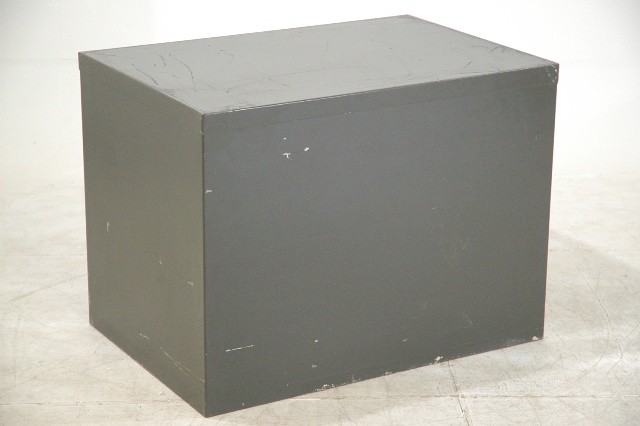This photograph features a plain gray rectangular crate or box, which appears to be constructed from painted wood rather than metal. The box is characterized by its solid gray color, with scattered white dings, chips, and scrapes that give it a slightly distressed look. Notably, the surface bears multiple scuff marks and scratches, particularly noticeable around the bottom and top edges. The crate is wider than it is tall and even less deep, emphasizing its squat proportions. It is placed on an off-white tiled floor, which resembles cement with faint lines that mimic a brick pattern. The background includes walls that are dark cream with a hint of blue.